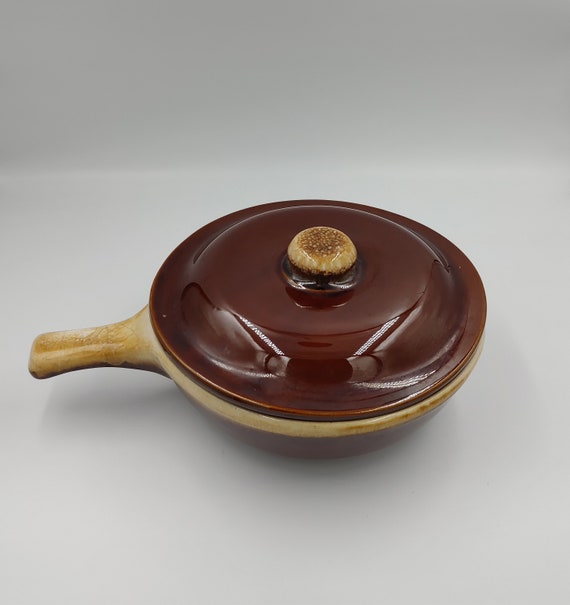The image depicts a ceramic pot with a predominantly brown, glazed lid that has a shiny, reflective surface. The lid features a circular shape with a small, round knob on top, resembling a hamburger bun in appearance due to its tan with a dark brown tip. The pot's handle is short and situated on the left side, blending into the background. The body of the pot transitions in color from white and off-white to yellow and brown. It stands on an off-white counter against a dark gray background that contrasts with the light reflecting off the glazed lid. The intricate details of light reflections and color variations give the pot a distinctive and visually appealing look.